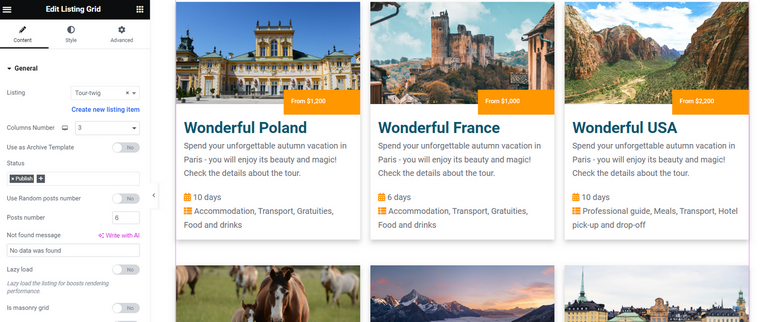An image showcasing an interface on a travel website is observed. The left side of the interface features a menu with options such as "Edit Listing Grid," "Contact," "Style," "Advanced," "General," "Listing," and "Tour Twig" accessible via a dropdown menu. Additional settings include "New Listing Item" and "Column Numbers" set to three, also with a dropdown menu. "Use Archive Template" is set to 'no,' while the status indicates 'publish.' The option to "Use Random Post Numbers" is also set to 'no.' The field for "Post Number" is set to six, but a message states, "No data was found." The "Lazy Load" option, which can boost rendering performance, is toggled off, and there is a reference to a "Masonry Grid" layout though the spelling appears incorrect as "m-a-s-o-r-r."

On the right section of the interface, the display shows travel listings arranged in two rows, though only the first row is fully visible. The first listing, titled "Wonderful Poland," advertises trips starting from $1,200 and highlights the opportunity to spend an unforgettable autumn vacation in Paris, enticing visitors with promises of enjoying its beauty and magic. It invites users to check details about the tour, which includes a ten-day itinerary covering accommodations, transport, gratuities, food, and drinks. The second visible listing is titled "Wonderful France."